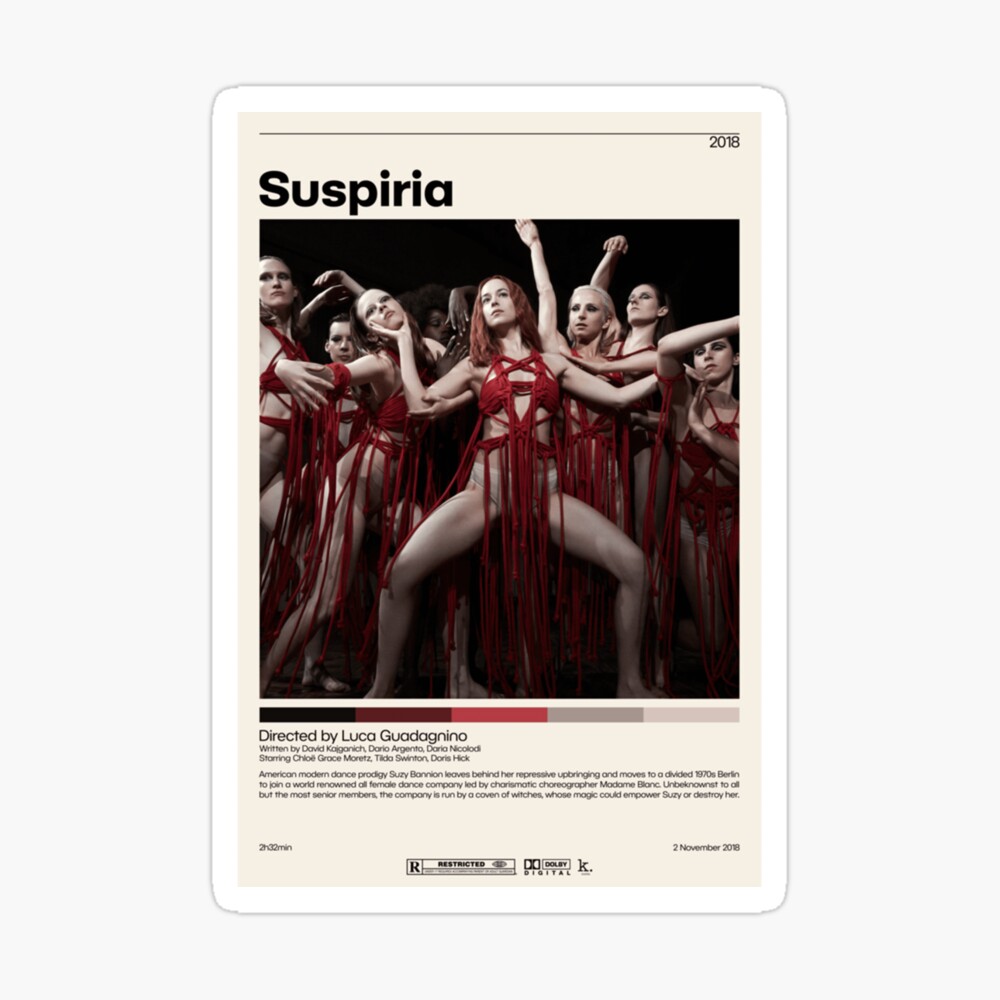The image is a vertical poster likely promoting the film "Suspiria," directed by Luca Guadagnino. Dominating the center of the poster is a provocative photograph featuring scantily clad women, presumably dancers, wearing white or beige underwear and red strappy bras or yarn-like cloth, with strings hanging down. These women are intertwined, posing against a backdrop filled with a mix of black, brown, red, gray, and light pink hues. The central figure appears to have red hair, with another blonde-haired woman behind her. The poster, enclosed in a white rectangle with a beige inset, prominently displays "Suspiria" in black letters at the top, along with the director's name and the year 2018. Various logos, including Dolby Digital, are visible at the bottom, along with an 'R' rating, further indicating that it's an advertisement for a movie.